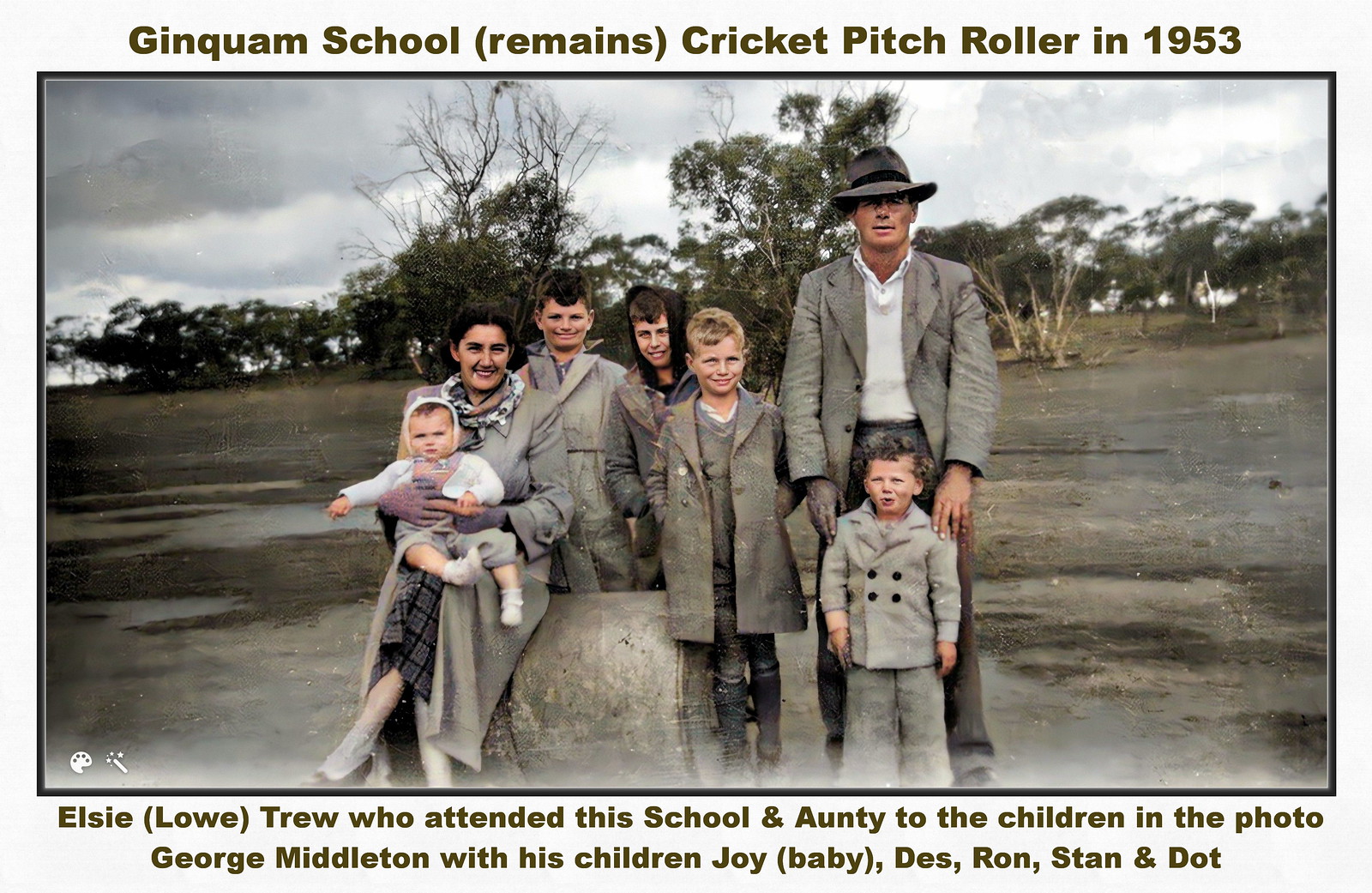This detailed photograph, likely restored and colorized from its original black-and-white version, captures a family scene from 1953, described in a newspaper-style caption. The photo shows George Middleton standing with his wife, holding a baby named Joy, alongside their other children: Des, Ron, Stan, and Dot. Also mentioned is Elsie Lowe Trew, who attended Ginnquam School and is the aunt to the children. The entire family, dressed in gray overcoats and appearing slightly worn from outdoor elements, pose in an outdoor setting with a cloudy sky and trees in the background. The father, George, wears a gray hat and places his hands on one of the children's shoulders. The composition hints at them sitting on or near a tree stump or similar object in what appears to be a park or open area with sparse foliage. The text above the photo mentions Ginnquam School remains and a Cricket Pitch Roller in 1953, indicating a historical connection to the location. Despite the dated attire and setting, the photograph's coloring and clarity suggest it has been retouched, possibly giving it a more contemporary appearance than its original era.